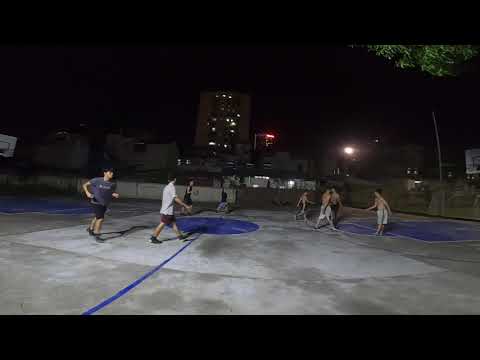This image captures a nighttime scene of eight young men, likely in their late teens or early 20s, engaging in a game of basketball on an outdoor park court. The court features a distinctive design with a central blue circle and surrounding lighter gray squares, while the outer rim comprises darker gray squares. The game appears to be a four-on-four matchup, with one team, the "skins," playing defense without shirts, and the other team, the "shirts," bringing the ball up to half court. 

In the background, a tall rectangular building with at least eight or nine floors is partially illuminated, with about a third of its windows lit. Adjacent to this building is another structure, which features a red sign at its top. A tree branch is visible in the top right corner of the frame, adding to the urban nighttime atmosphere. The court’s concrete surface is clearly illuminated by the limited ambient lighting, highlighting the blue lines delineating the playing area and out-of-bounds zones.